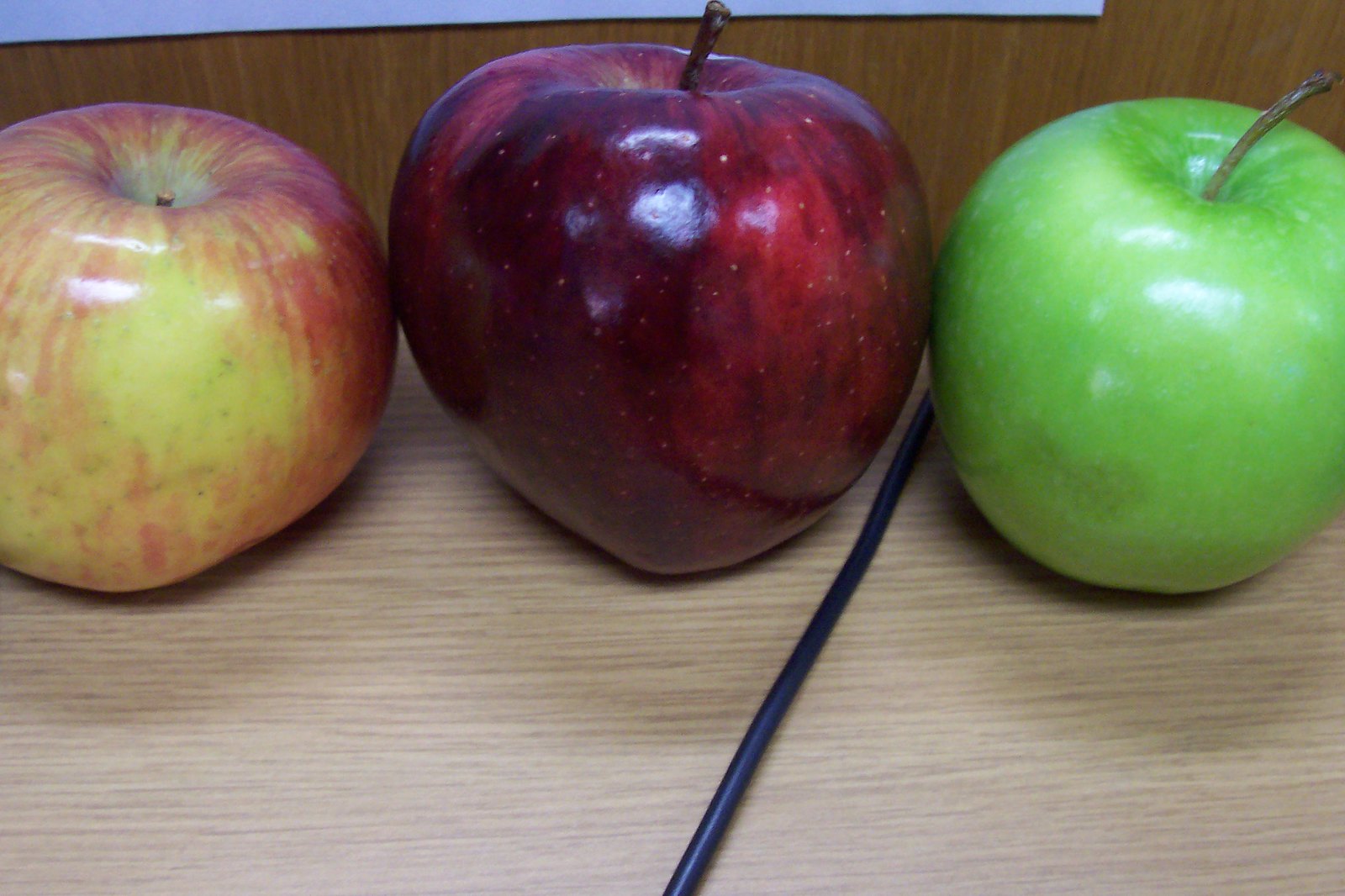The close-up image features three distinct apples, each with unique colors and characteristics, arranged in a row on a wooden or wood-like surface. 

On the far left, there is an apple with a gradient blend of reddish and yellow hues, displaying a slightly smaller size compared to its neighboring fruit. 

In the middle, a larger apple stands out with a uniform, deep red color, exuding a rich and glossy surface. 

To the far right, the final apple is bright green and slightly smaller than the central dark red apple. 

All three apples appear exceptionally shiny, suggesting they are fresh and well-polished. A black wire runs between the dark red apple and the green one, adding an intriguing element to this otherwise natural setting.